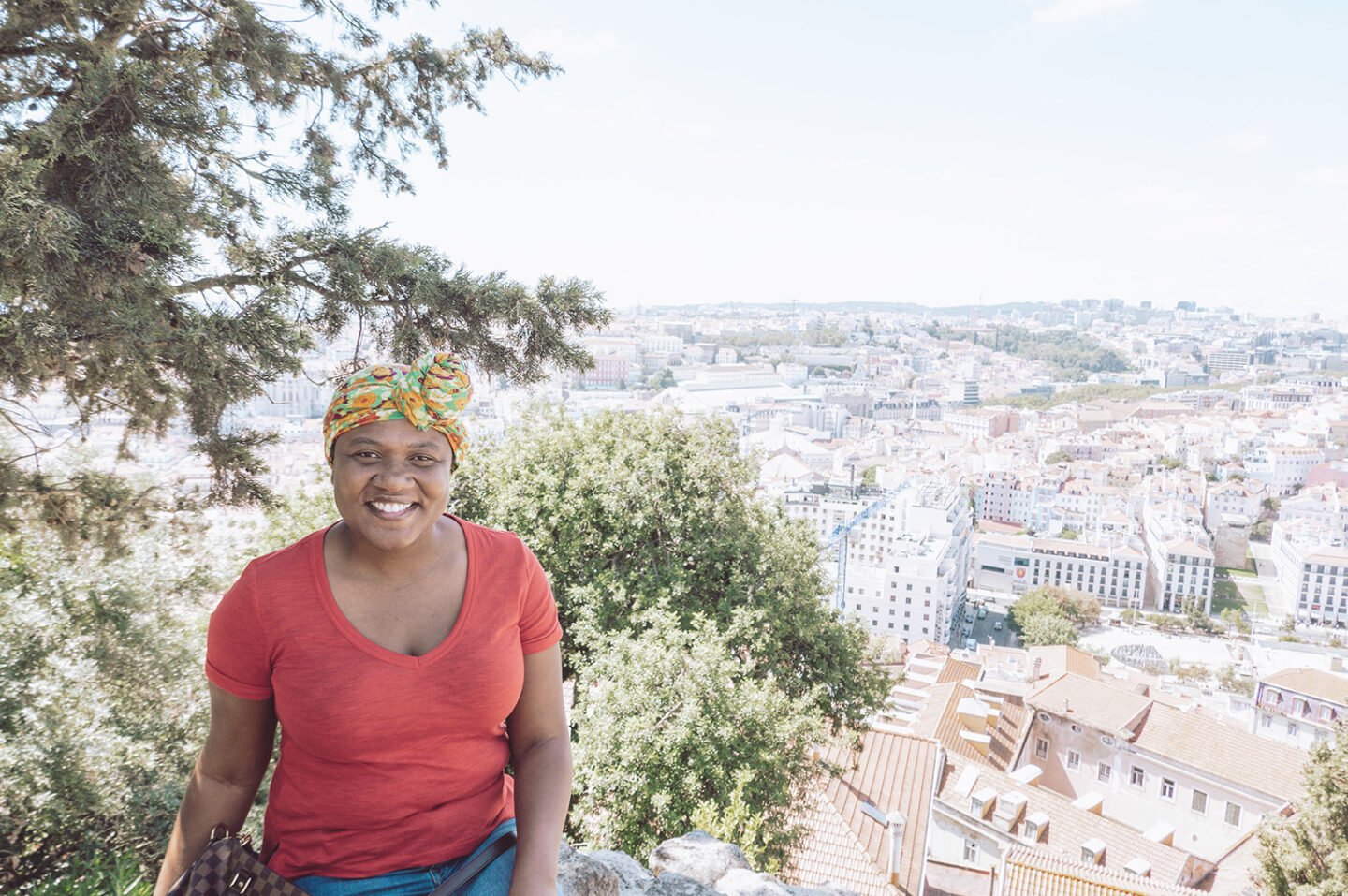A very young woman with light brown skin sits to the left of the foreground, smiling broadly at the camera. She wears a red scoop neck T-shirt with short sleeves, revealing the top of her jeans, and a colorful headscarf in orange, green, and white, tied into a bun on the right side of her head. She's seated on an outcropping of rocks, barely visible in the photograph, amidst summer greenery including trees and bushes adorned with small white flowers. To the upper right of the frame is a tree, while a corner of a house's roof and a wooden walkway can be seen to the right of the bush. The background stretches out to reveal a sunlit cityscape with industrial buildings, apartment complexes, and red roofs, gently dropping away from the hillside she sits on. The entire scene is bathed in bright sunlight, suggesting a warm, tranquil day.